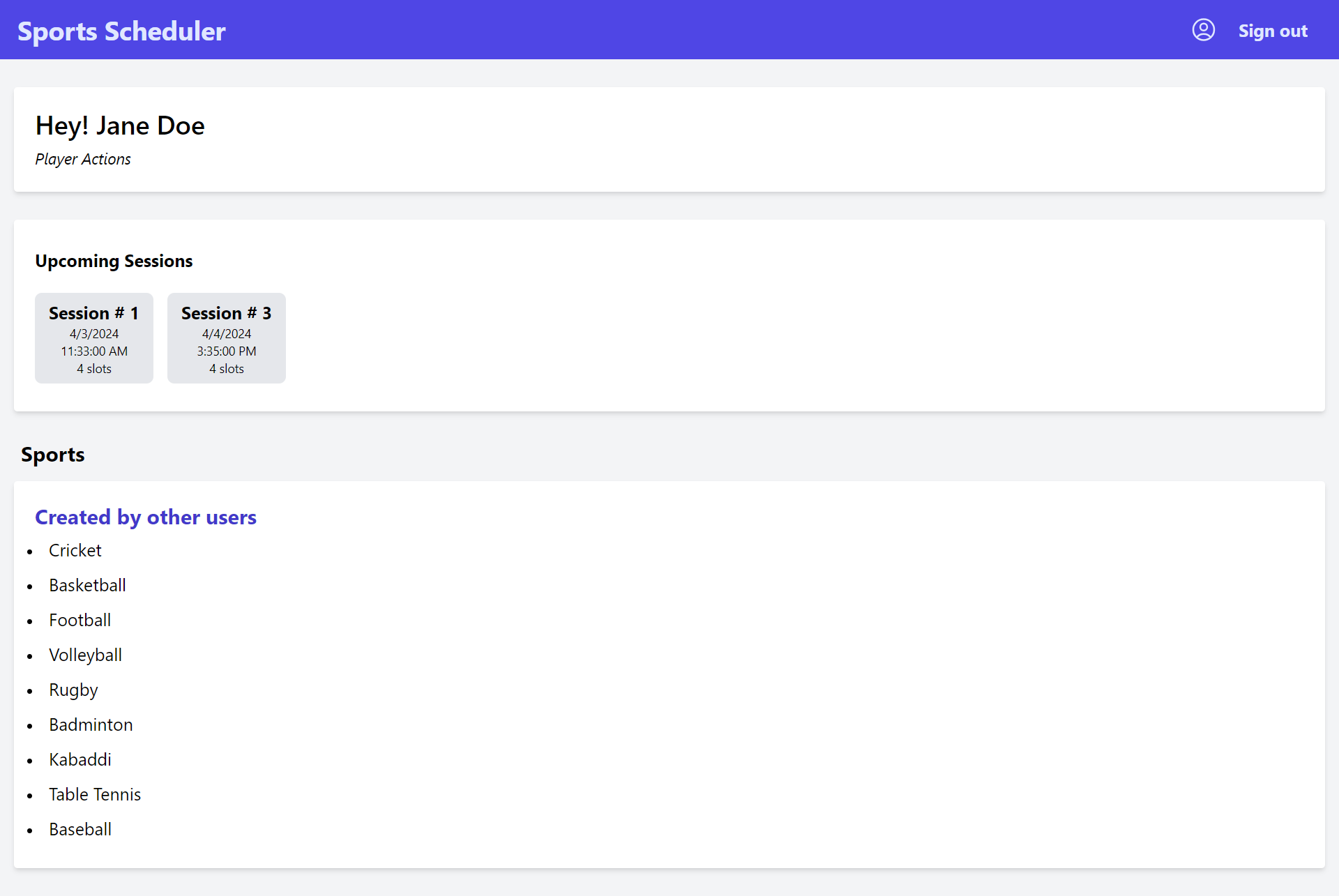Caption: 
A screenshot showcasing the user interface of the "Sports Scheduler" portal, where an individual is signed in (indicated by the "Sign Out" option). The interface greets the user with a "Hey Jane Doe" message. Below this greeting, it lists upcoming sessions: 

- Session 1: April 3, 2024, at 11:33 AM with four available slots.
- Session 3: April 4, 2024, at 3:35 PM with four available slots.

The portal also features a section titled "Sports Created by Other Users," highlighting various bullet-pointed sports options including cricket, basketball, football, volleyball, rugby, badminton, kabaddi, table tennis, and baseball. The titles "Sports Scheduler" and "Created by Others" are prominently displayed in bright blue, while the general text uses a basic black font, creating a clear and user-friendly design.